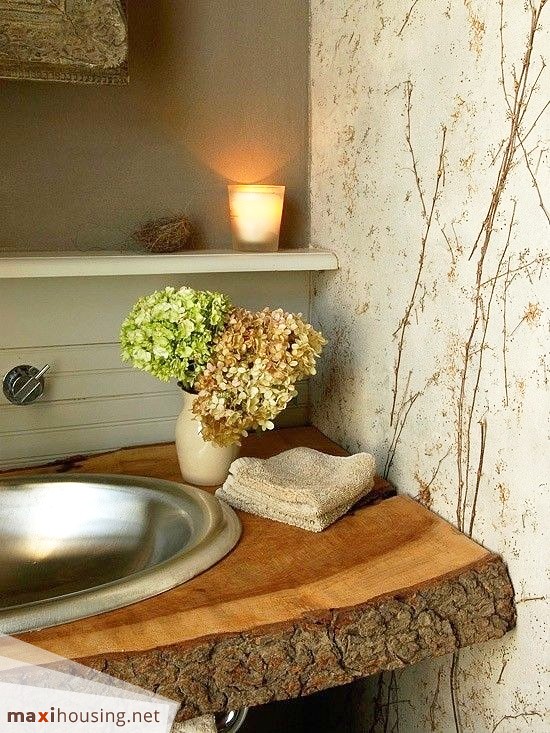The image portrays a bathroom scene dominated by a vertically oriented composition, approximately 20-30% taller than it is wide. Central to the image are two distinct walls. The left wall forms the right side of a bathroom sink area, with a unique sink counter fashioned from a cross-section of a tree trunk, showcasing the natural bark on the near edge and well-defined wood grains running horizontally. The steel sink, partially visible on the left, features a faucet handle rising above it. Placed on the wooden counter are a couple of washcloths and a vase containing predominantly green flowers interspersed with some browning, wilting ones. Above this counter lies a small shelf holding a candle.

The contrasting right-hand wall presents a decorative design. It is predominantly off-white, embellished with vertical, gold lines resembling sticks, scattered in a loosely parallel arrangement. These golden accents contribute a subtle yet striking visual texture to the wall.

In the lower left-hand corner of the image, the website "maxi-housing.net" is inscribed, suggesting a possible association with the depicted interior.